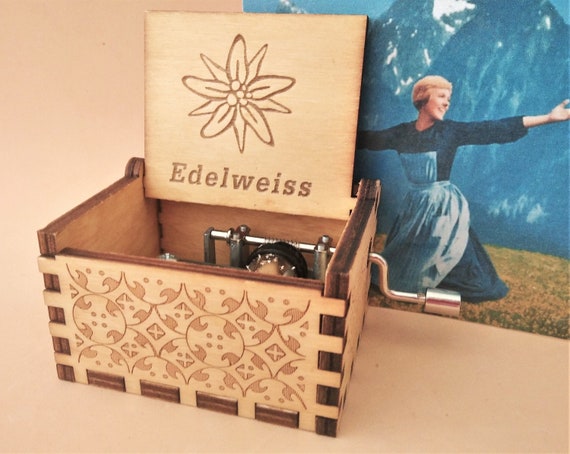The photograph captures a nostalgic scene reminiscent of "The Sound of Music," featuring Julie Andrews in her iconic role. She stands on a high German mountain, with vast, dark, and snow-capped peaks behind her, and a field of yellow flowers at her feet. Julie sports a dark blue dress with a white apron, short blonde bobbed hair, and her arms stretched wide, as if singing or dancing with joy. In the foreground, a detailed wooden music box is prominently displayed. This light brown music box features elegant darker trim along its edges and intricate carvings, including a flower and the word "Edelweiss" etched on its lid. The box is open, revealing its inner mechanisms and a silver metal handle on the right side that winds it. The photograph has a slightly dated, muted color palette, adding to its vintage charm.